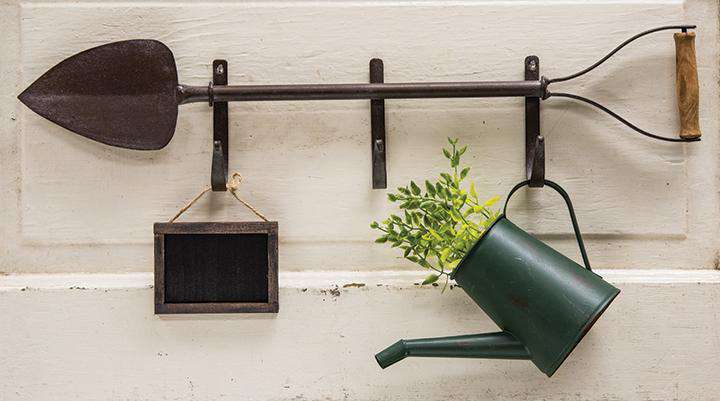The image depicts a set of gardening tools neatly organized on a white, weathered wall with a textured surface. The wall features a raised rectangular area and a thick raised trim at the bottom, adding to its rustic charm. Three metal, hook-shaped brackets are mounted on the wall. Resting across these brackets is a shovel with a dark-colored, teardrop-shaped metal scoop and a wooden handle. Directly below this, a green watering can is hung from one of the bracket hooks, with a plant growing out of it, adding a touch of greenery to the arrangement. Additionally, a small rectangular chalkboard with a wooden frame dangles from another bracket, completing the scene with a functional yet decorative element.